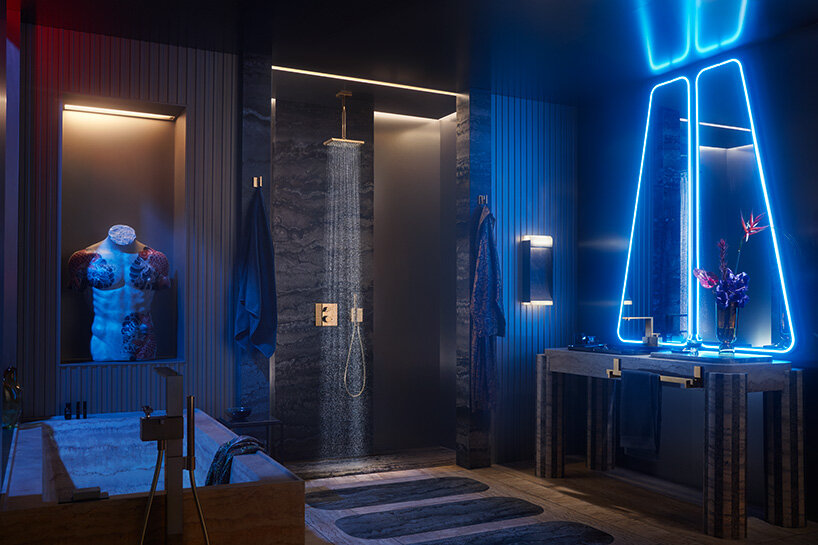This photograph depicts a stylish, modern bathroom with dramatic and dark lighting. Dominating the right side of the image is a sink area featuring two geometric, almost rhombus-shaped mirrors with bright blue neon lights outlining their borders. A plant with a vibrant red flower adds a hint of nature to the sleek setting. The sinks appear to float with no visible piping underneath. Adjacent to this area is an open shower, centrally positioned in the room, showcasing a ceiling-mounted, square showerhead emitting rain-like water.

On the left side of the image, a contemporary square bathtub appears to connect with just one wall, enhancing the room's avant-garde design. Behind the bathtub, a built-in depression in the wall houses a backlit bust statue or mannequin torso, adorned with what seem to be traditional Yakuza-style tattoos of koi fish, adding an artistic element to the space. A bathrobe and towel are neatly hung near the entryway. A rug placed in front of the shower completes the setup, making it a perfect blend of modern luxury and artistic flair.